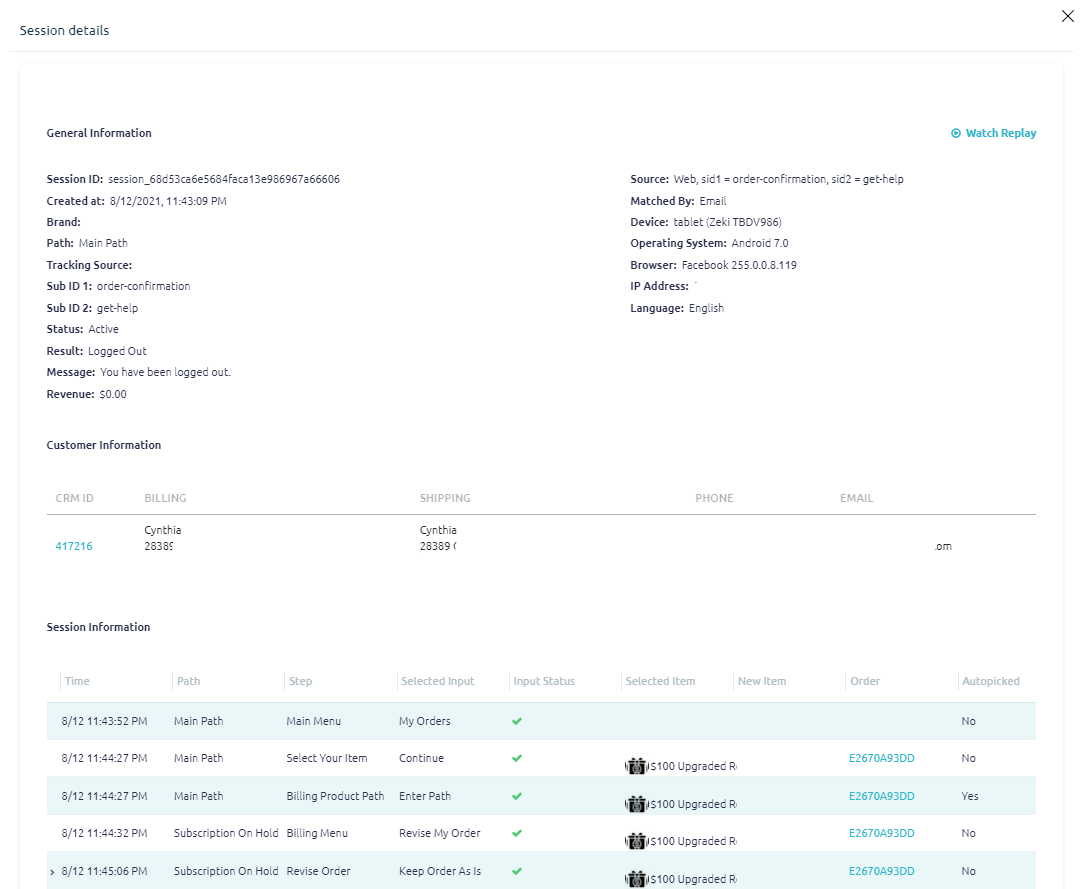This image, captured from someone's cell phone, displays a detailed session details screen. At the top, there's a header labeled "Session Details." Below, a faint gray line outlines a rectangular section that organizes the information.

The left side of the screen begins with the heading "General Information," followed by "Session ID," which includes a long string of alphanumeric characters prefixed by "session_." Directly below, it indicates the creation date and time: "8/12/2021 11:43:09 PM."

The next section lists various attributes: "Brand" is left blank, "Path" is labeled as "main path," "Tracking Source" is also blank, "Sub ID 1" reads "order-confirmation," and "Sub ID 2" states "get-help."

Further down, the status of the session is "Active," the result is marked as "Logged out," accompanied by a message stating, "You have been logged out."

Towards the bottom, the section titled "Session Information" comprises a chart. The chart headers include "Time," "Path," "Step," "Selected Input," "Input Status," "Selected Item," "New Item Order," and "Auto Pick." The rows alternate in color between blue and white and contain green check marks under the "Input Status" column, indicating completed steps in the session.